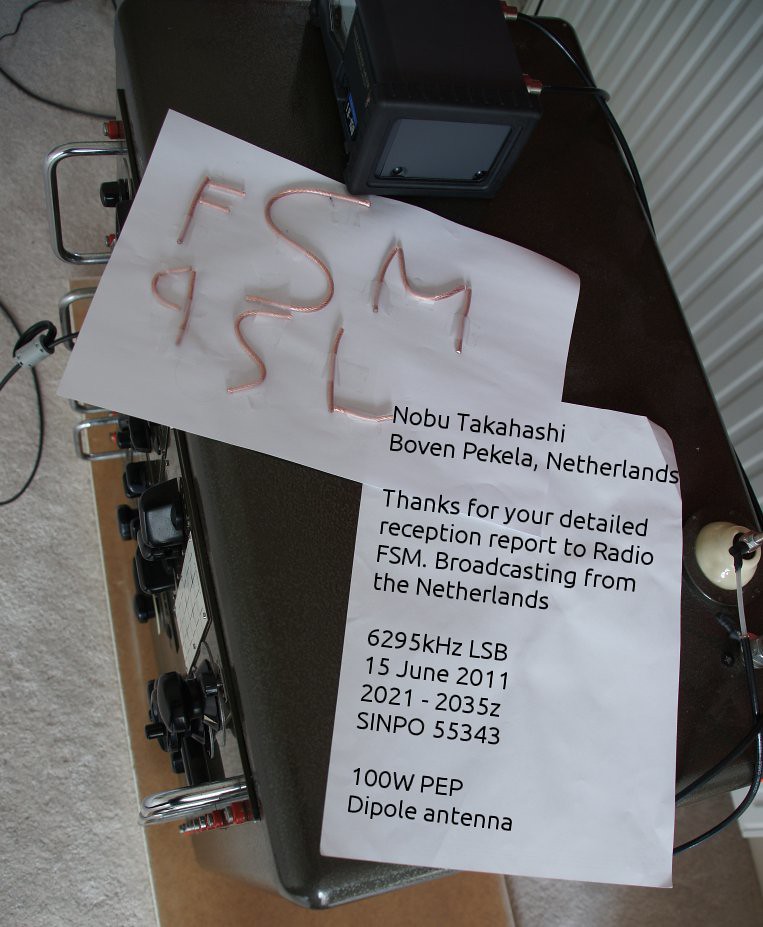The photograph captures a detailed scene inside a room, focusing on a safe lock box adorned with two pieces of paper. Metal handles protrude from the left side of this intricate contraption, which is dotted with numerous knobs. On top, one piece of paper prominently displays copper wires bent to spell out "FSM QSL." Adjacent to this, a printed receipt reads: "Nobu Takahashi, Boven, Pekkela, Netherlands. Thank you for your detailed reception report to Radio FSM, broadcasting from the Netherlands, 6295 kHz LSB, 15 June 2011, 2021-2035 Z, SINPO 55343, 100W PEP, Dipple Antenna." The scene is meticulously arranged, with emphasis on the papers and the unique details of the machine.